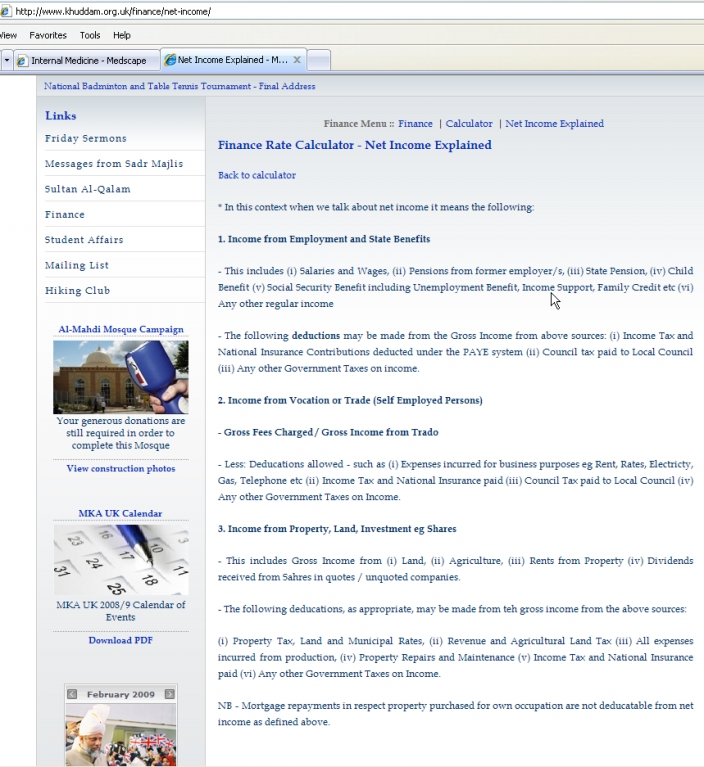The image is a vertically oriented rectangle, displaying a webpage viewed through the Internet Explorer browser. The browser has two open tabs, with the active tab titled "Net Income Explained" and the inactive tab labeled "Internal Medicine Medscape." 

At the top of the browser, a gray banner spans across the screen, featuring menu items: "View," "Favorites," "Tools," and "Help." 

The main portion of the webpage is divided into sections. On the left side, a vertical sidebar lists various links: "Links," "Friday Sermons," "Messages from Sader Mejiles," "Sultan Al-Kalam," "Finance," "Student Affairs," "Mailing List," "Hiking Club," "Calendar," and "Mosque Campaign."

Dominating the main content area, the header reads "Finance Rate Calculator," with the primary title "Net Income Explained" highlighted in blue. Below, a link allows users to navigate "back to calculator." 

The descriptive text states: "In this context, we will talk about net income," and elaborates further with sections detailing different sources of income:
1. "Income from employment and state benefits."
2. "Income from vocation or trade."
3. "Income from property, land, investment, i.e., shares."